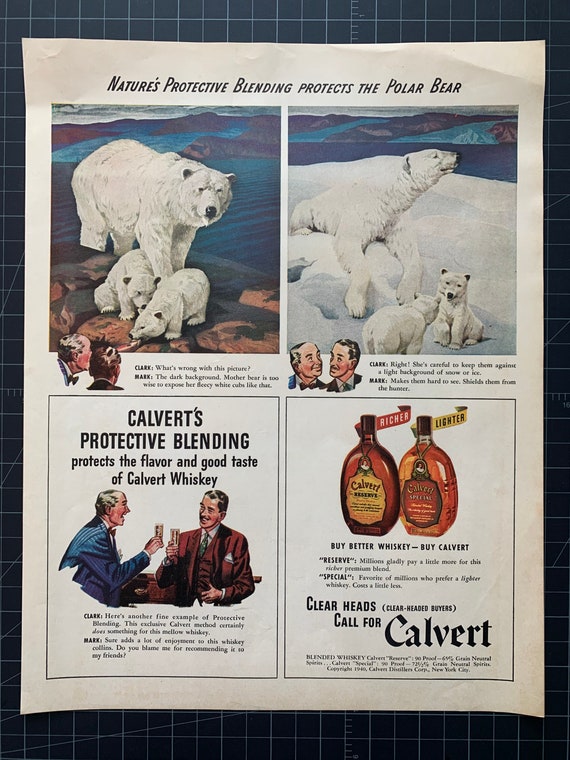The image captures a page, possibly from a mid-century magazine or flyer, laid flat on a dark measuring table. The page is divided into four quadrants. The top two quadrants feature a mother polar bear with her two cubs; the left image shows them on dry land, while the right image depicts them on an icy terrain. Below each image, there is text and headshots of two men, Mark and Clark, who appear to be discussing the contrasting scenes. The text above these images reads, "Nature's Protective Blending Protects the Polar Bear."

The bottom left quadrant shows two men enjoying glasses of Calvert whiskey, raising a toast. The accompanying text highlights the quality of the whiskey, stating, "Calvert's Protective Blending Protects Flavor and Good Taste of Calvert Whiskey." The bottom right quadrant directly advertises Calvert whiskey, displaying two bottles with a tagline beneath them that emphasizes the product's appeal: "Clear Heads Call for Calvert." The advertisement juxtaposes the protective blending concept for both the bears and the whiskey, creating a thematic connection.